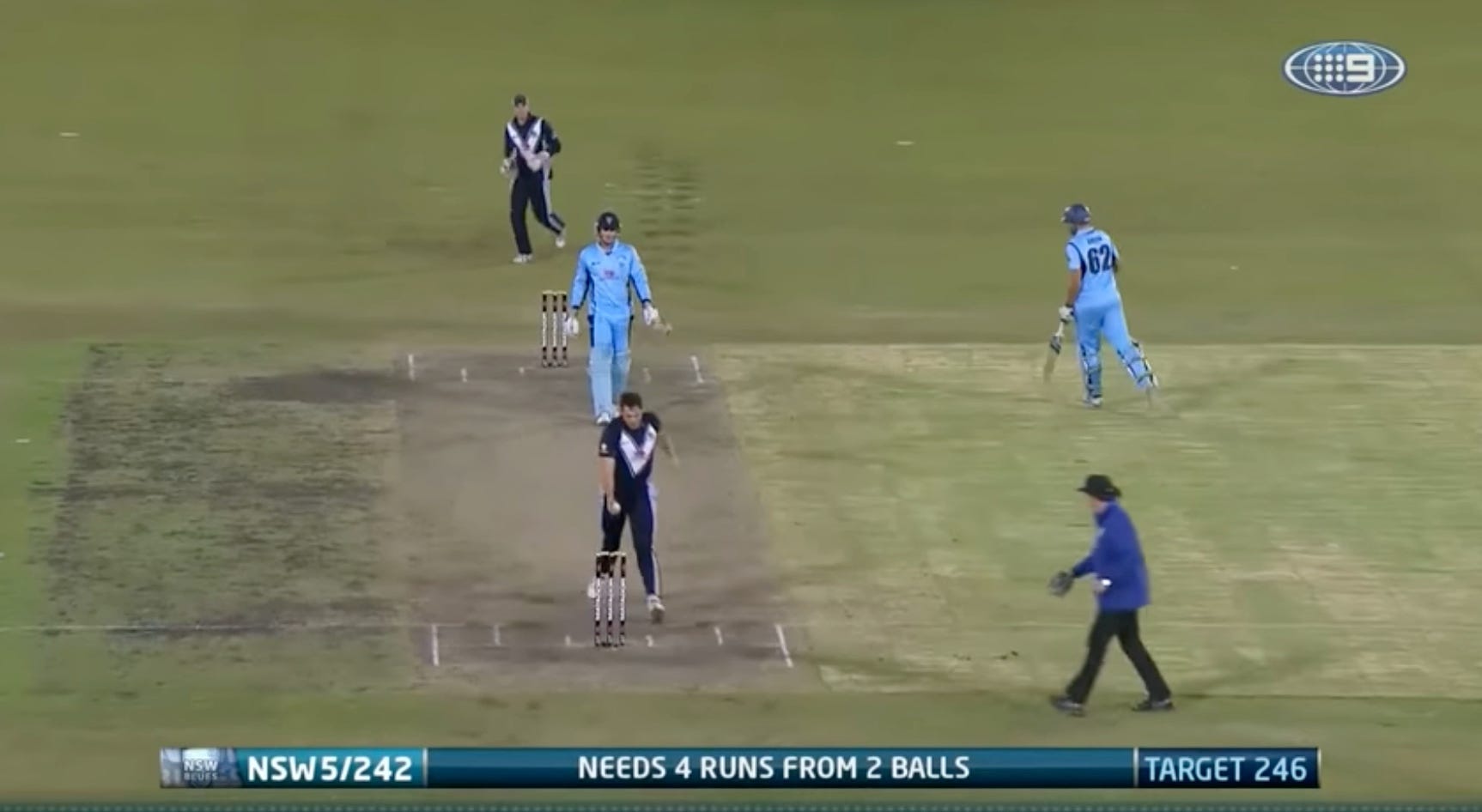The image depicts an intense moment in a cricket match with a scoreboard overlay at the bottom of a TV screen, displaying in white letters on a blue background: "NSW 5/242," "Needs 4 runs from 2 balls," and a "Target 246." The field appears to be covered in a flat, green surface, resembling a rug, rather than natural grass. There are five players visible: 

- The bowler, dressed in a black uniform with a white V on the chest, is holding a ball in his right hand.
- Standing behind the bowler is a fielder in a light blue uniform and white gloves, with a cap on his head.
- In the upper right section, a player with a blue uniform and the number 82 on his back is running while carrying a cricket bat.
- On the left side, another player in a black uniform with a white V appears to be running to the left.
- In the lower right corner, a person who could be an umpire or coach is seen wearing a blue jacket and black pants, walking from right to left, possibly to confer with the bowler.